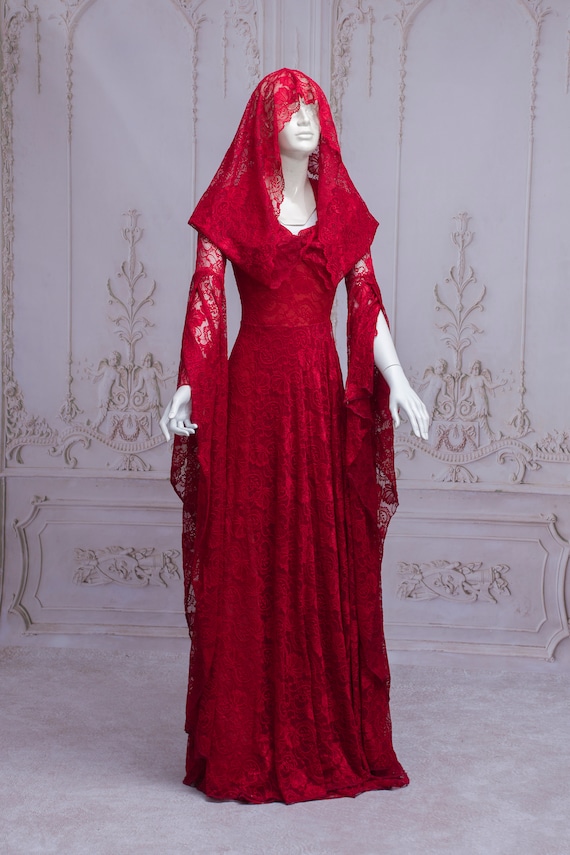In this detailed photograph, a white female mannequin stands against a strikingly regal backdrop. The mannequin is a lifeless, sleek, and tall figure made of plastic, exhibiting a stark contrast to the rich background. It wears a stunning red dress made entirely of lace, which covers it from head to toe. The dress has long, flowing sleeves, which, while slit up to the elbow, cascade down gracefully to about the knees. A matching lace veil drapes elegantly over the mannequin's head, extending down over the shoulders and obscuring the eyes. The vivid red lace of the dress and veil pops dramatically against the mannequin's white form, drawing the viewer's attention immediately. 

The background features an ornate wall, reminiscent of an opulent French apartment or museum. The wall is adorned with intricate 3D carvings and designs, possibly of cherubs or angels, embodying a style akin to Art Nouveau. This elaborate setting, with its detailed relief work of flowers and children, adds an additional layer of luxury and refinement to the scene, emphasizing the mannequin's elegant attire.